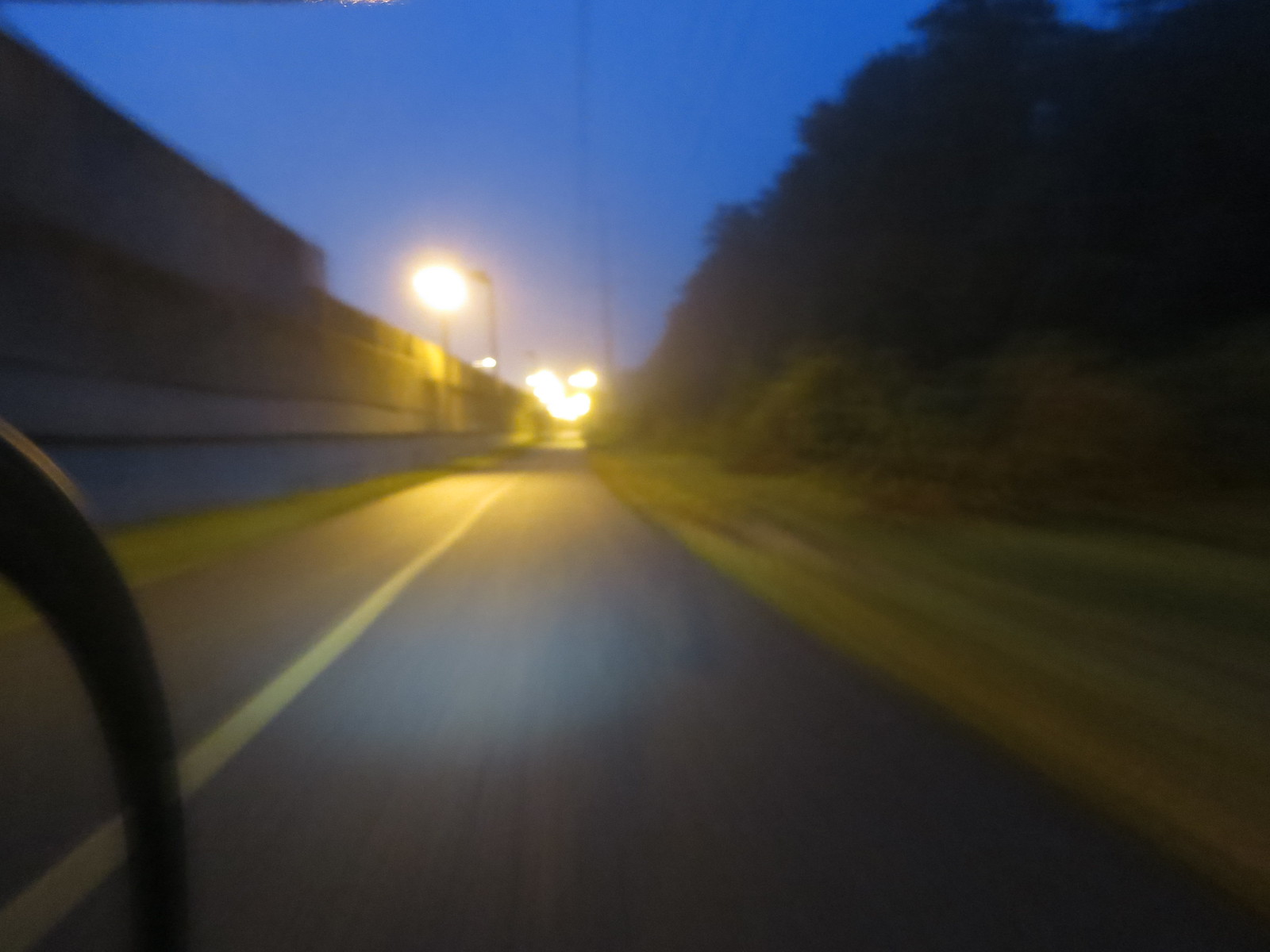The image captures a private service road branching off a highway, characterized by its solid yellow center line. Taken from the interior of a vehicle, the photo includes a partial view of the car's dashboard. A prominent retaining wall dominates the left side of the road, while the right side features a manicured lawn with trees and bushes dotting the landscape. The day appears to be transitioning into evening, as evidenced by the rich blue sky and the activation of overhead street lights. High electric wires run parallel to the road, emphasizing the infrastructure present in the area. The scene is illuminated by multiple bright lights lining the road, enhancing visibility as dusk approaches.